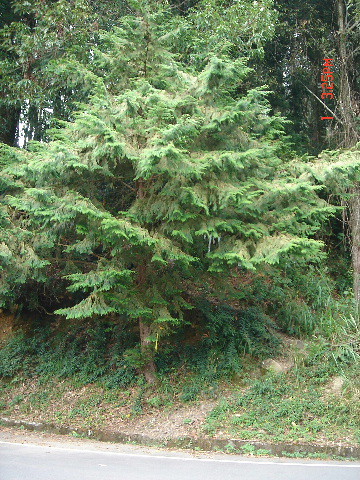This outdoor daytime photograph, likely taken with an old camera, captures a roadside scene marked by a timestamp reading "1 325 p.m." in red print on the upper right corner. The small rectangular image, approximately four inches high and three inches wide, shows a narrow strip of gray paved tarmac at the bottom with a white stripe. A brown cement curb borders the road, leading to a sloping hill covered in dirt, small patches of grass, and bits of foliage sprouting from the curb.

Dominating the middle of the hill is a large, bushy coniferous tree with predominantly green foliage accented by whitish tips, and a hint of light tan within. Beyond the prominent tree, the backdrop transitions into a dense forest with thin, vine-entangled trees, through which patches of white sky can be glimpsed. There's also a small brown area at the tree's base, potentially suggesting a walkway leading into the woods. The details converge to paint a vivid picture of a serene, slightly wild roadside edge merging into a forest.